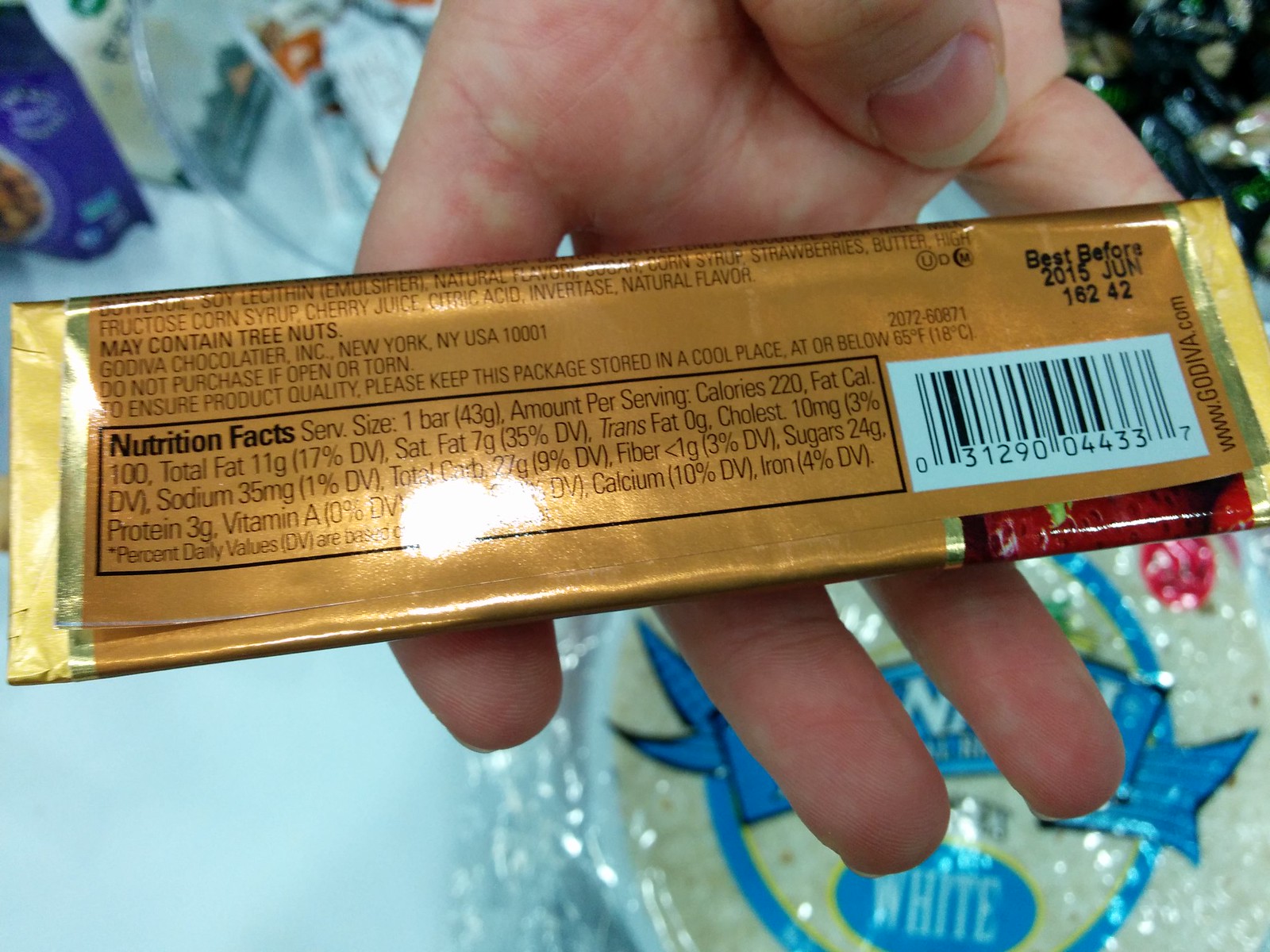This indoor color photograph provides a detailed close-up of a Godiva chocolate bar being held in a partially visible right hand, likely a white female's. The bar is upside down, displaying the gold-wrapped back of its label. Dominant black printing covers the label, including a prominent Nutrition Facts section outlined in a black rectangle on the lower half. Above this section, it warns in all caps that the product "MAY CONTAIN TREE NUTS." In the bottom right corner lies a white barcode with black stripes (0 3 1 2 9 0 0 4 4 3 3 7), and above it, the Best Before date reads "2015 JUNE" with an additional code "J6242." The vertical "www.godiva.com" is also printed in capital letters near the barcode. The hand, clutching the bar with fingers extended and thumb curled inward, emerges from the top of the image. The background features a white surface; the lower right corner contains a package of white tortillas, while the upper left hints at a glass mixing bowl and other indistinct items.